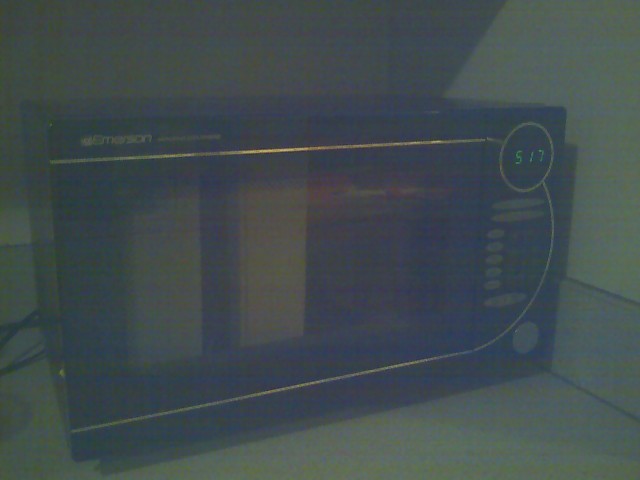This color photograph, taken in very dim, low light, showcases a blurry, grainy image of a microwave on a countertop. The overall color palette appears dull with a greenish tint. The microwave itself is predominantly black with silver accents, including a horizontal silver lining and a circular silver rim around the display on the right side. The display shows the number 517 in bright green. Below the display is a series of horizontal buttons and a round button at the bottom. The top left corner of the microwave has a barely discernible logo, possibly reading "Mason." The surrounding environment suggests a kitchen setting with a dark, slanted wall behind the countertop, possibly indicating an attic roof. The left side of the image is lighter, with what appears to be a cord coming out and a smaller shadow near the bottom left corner.